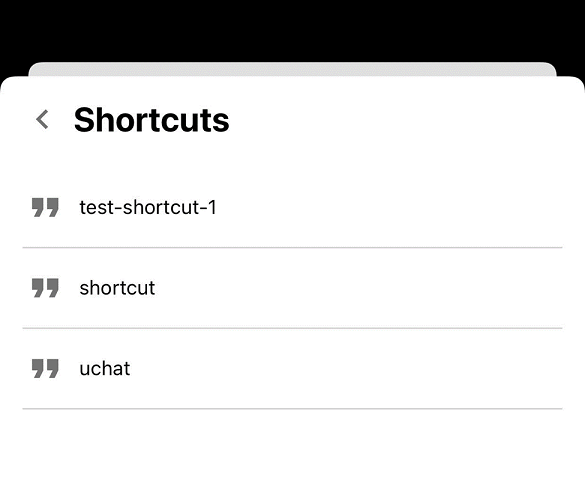The screenshot appears to be taken from a tablet device and features an application interface. The screen has a black background, and prominently displayed in the center is a white tab with the heading "Shortcuts" in large, bold black text. Below the heading, there are three distinct entries:
1. "test-shortcut-1"
2. "just shortcut"
3. "uchat"

Each entry is enclosed within quotation marks and listed on separate lines. Partially visible behind this "Shortcuts" tab, there seems to be a light gray edge of another page or box that is part of the app's user interface, although it is only faintly discernible and offers no additional context about the app's nature or functionality. The overall layout and design elements suggest it could be a common feature found in various applications.